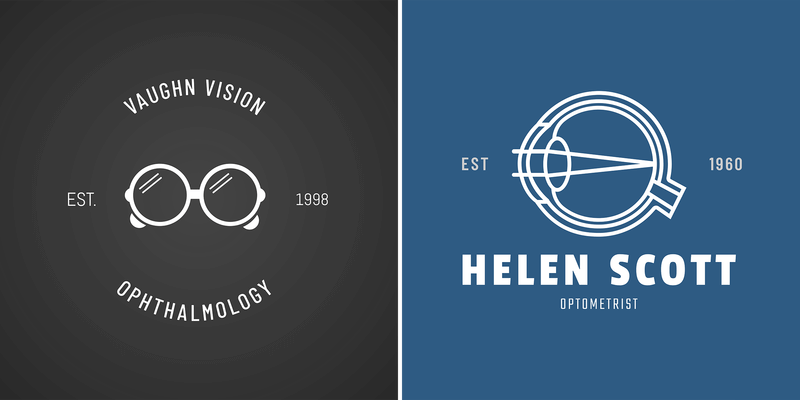This image features two adjacent graphic logo designs representing two distinct eye care professionals. 

On the left, a black background showcases white text and imagery. At the top, "Von Vision" is written in an arched fashion, mirrored by the word “Ophthalmology” at the bottom, both forming a circular design. Within this circle, there's a depiction of round eyeglasses, with "EST 1998" inscribed to the left and right of the glasses. This design symbolizes an ophthalmology practice established in 1998.

On the right, a blue background highlights a transparent diagram of an eyeball with light entering through the iris to the back of the eye. To the left of this diagram, it says “EST,” and on the right, “1960.” Below this, the name "Helen Scott" is prominently displayed in bold, uppercase white letters, with "Optometrist" in smaller white text underneath. This simple yet informative logo signifies an optometrist practice established in 1960.